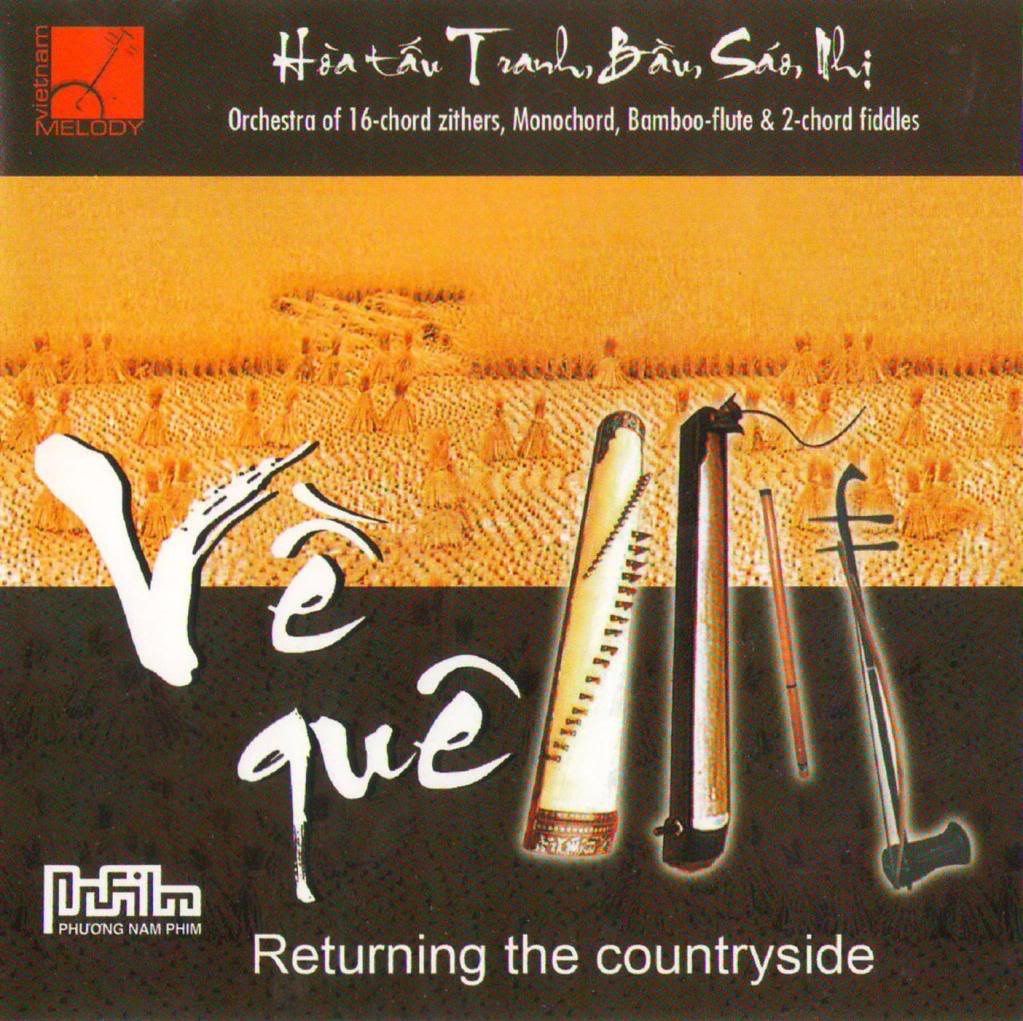This detailed infographic appears to be an advertisement for a Vietnamese concert or event titled "Vietnam Melody." At the top, a black banner showcases a red logo with an illustration of an old string instrument, alongside a calligraphy-style text in Vietnamese. Below this, white lettering announces "orchestra of 16 chord zithers, monochord, bamboo flute, and two chord fiddles." 

In the middle section, there is a faint, decorative image resembling a stage where several costumed people appear to be dancing. This image looks almost burned in or embroidered, adding to the traditional aesthetic. Beneath this, more calligraphy-like text spells out "Decay" in white font. 

Further down, images of four traditional instruments are displayed: one with several strings and a cylindrical shape, another cylindrical with a small tube at the top, a stringed instrument shaped like an axe, and a flute-like instrument. 

At the bottom of the image, it says "Returning the Countryside" in white letters on a brown background. Additionally, the image includes the phrase "Phu Thong Nam Phim" in white text on the bottom left corner, enhancing the cultural context and authenticity of the event being advertised.